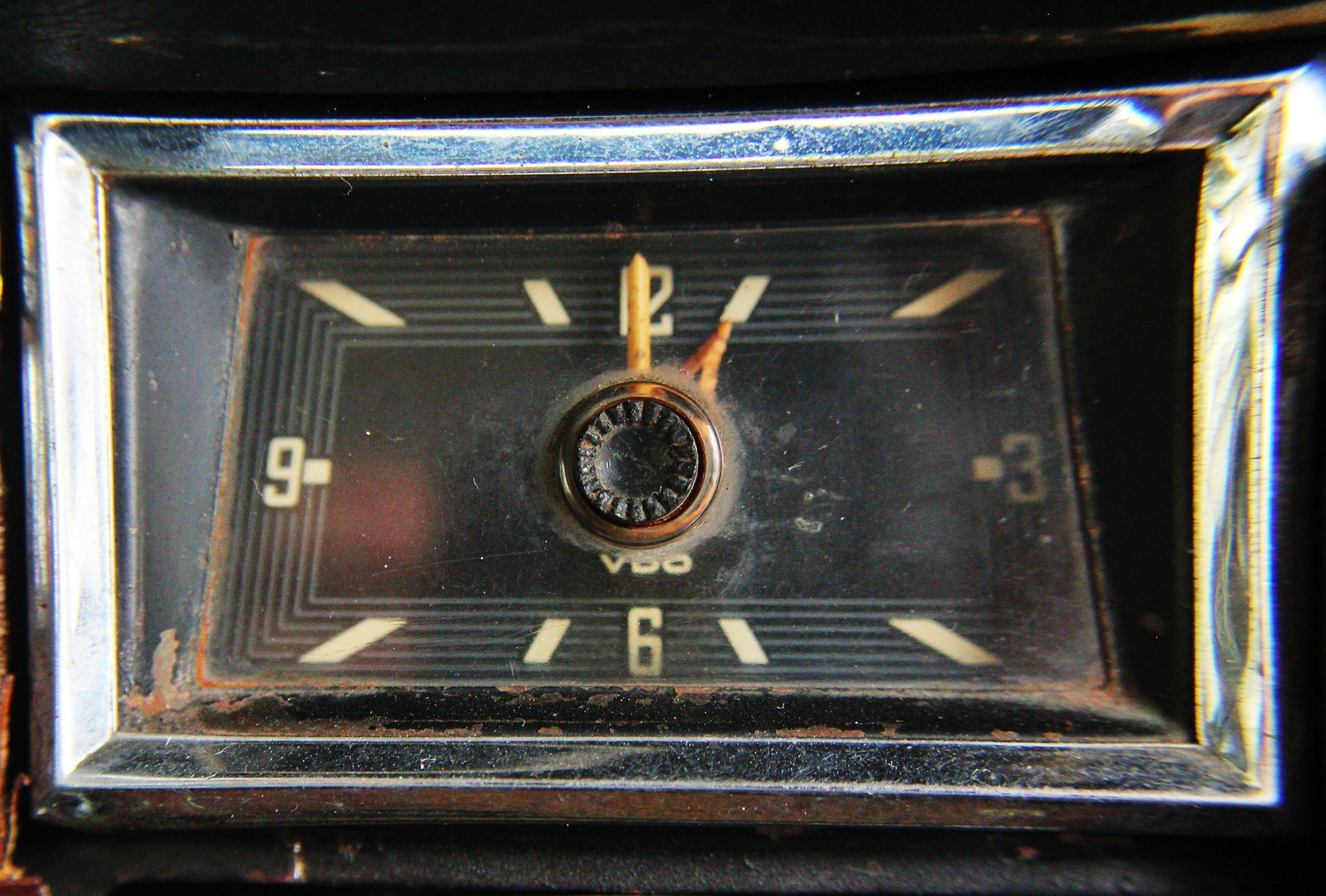This image showcases a vintage clock embedded in what appears to be an appliance, likely an oven, given its function as a timer. The clock features a silver-edged rectangular frame, lending an air of mid-century design. Prominently displayed are the numerals 12, 3, 6, and 9, with simple lines marking the other hours. At the center of the clock face is a black button, presumably for adjusting the dials. The age of the device is evident from the visible rust, wear, and buildup of grime. The time displayed is precisely 1 o'clock.